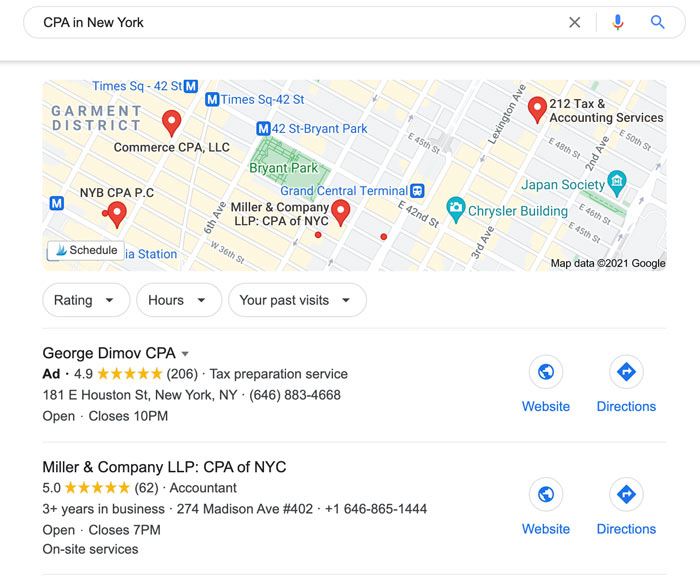The Google search results for "CPA in New York" are displayed on the page, featuring a detailed search interface that includes voice search functionality. At the top, there is an interactive map highlighting various CPA locations within the Garment District, providing visual context relative to landmarks like the Japan Society and the Chrysler Building.

The map showcases the positions of several CPA firms, including Commerce CPA, NYB CPA, Miller & Company LLP CPA, and 212 Accounting and Tax Services. Below the map, brief listings of CPA services appear, starting with a sponsored ad for George Dimov CPA. This ad presents a highly-rated tax preparation service with 4.9 stars, located at 181 East Houston Street, New York, NY. It includes clickable options for visiting the website or obtaining directions but is not shown on the map itself.

Additionally, Miller & Company LLP CPA is featured prominently with a 5-star rating and over three years in business. This firm is located at 274 Madison Avenue, Suite 402, and is visibly marked on the map.